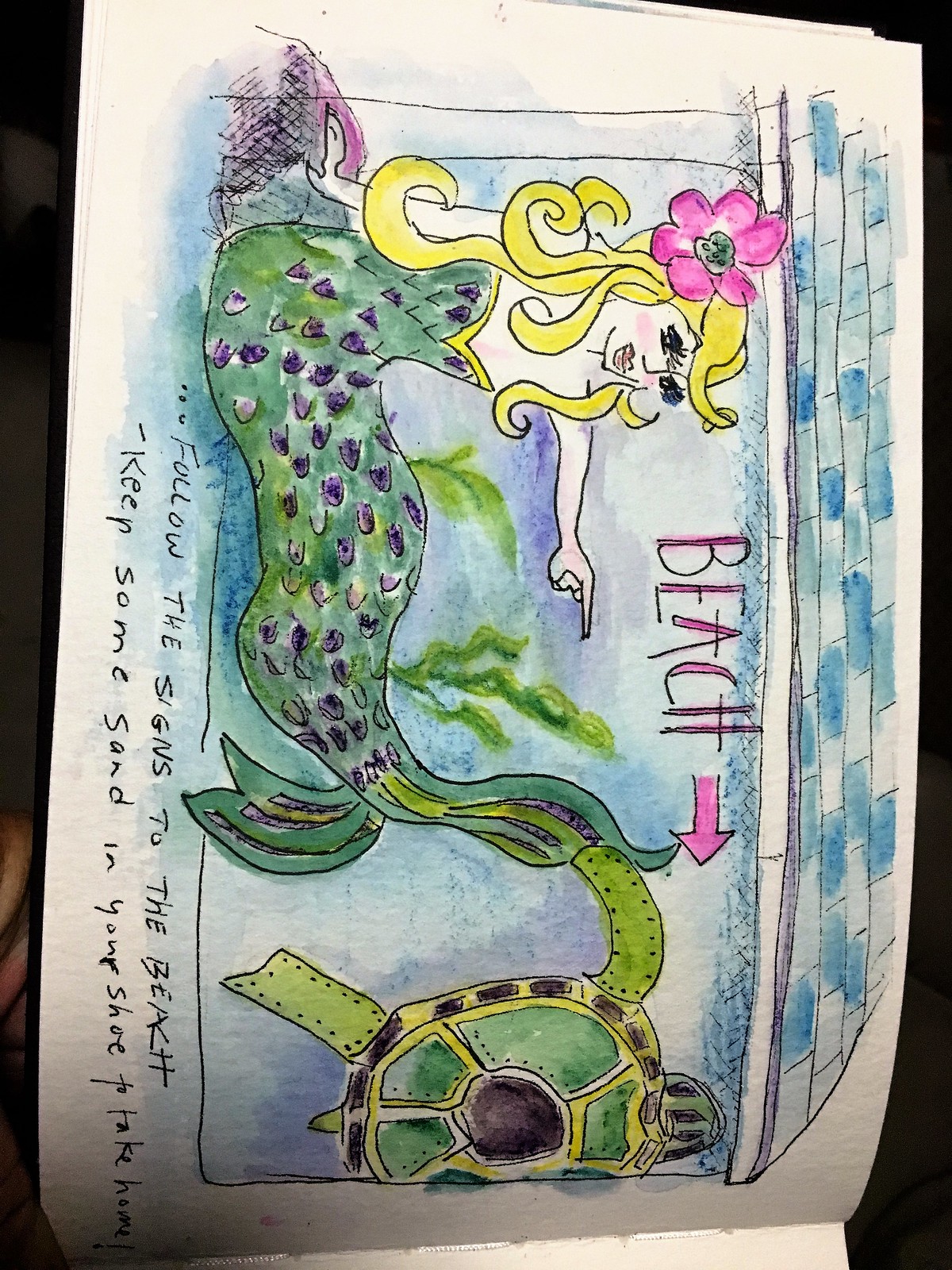This indoor color photograph captures a page from a sketchbook, turned 90 degrees to the right, detailing a whimsical scene with a mermaid and a sea turtle against a building backdrop. The mermaid, positioned with her torso at the top and her tail pointed downward, has flowing blonde hair adorned with a pink flower featuring a green center. Her vibrant green tail is decorated with purple scales. Her left hand points downward, her head faces to the right, and her expressive eyes are open. Below her, a green turtle is depicted from the top view, showing a green shell with a black spot at its center. The building behind them displays light blue and dark blue rectangles, representing its roof. 

The mermaid is accompanied by vertical pink lettering at the center of the page, spelling out "BEACH," with an arrow pointing to the right. To the left edge of the page, vertical text advises, "Follow the signs to the beach and keep some sand in your shoe to take home." The sea-themed background includes blue hues and a touch of seaweed, enhancing the aquatic ambiance of the imaginative illustration.